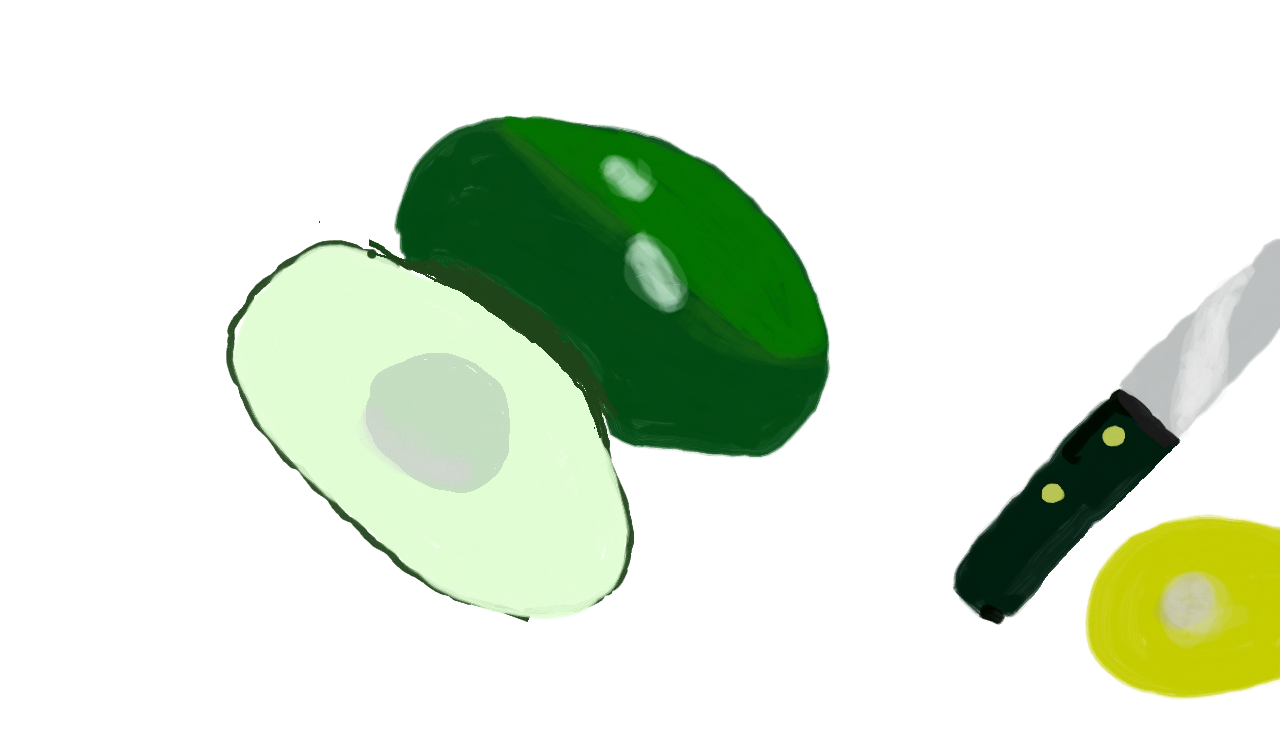The image, which appears to be created using a program like Microsoft Paint or possibly hand-painted, is set against a white background and depicts a still life scene with distinct detailed elements. On the left side, there is an avocado featuring a dark green exterior and green flesh, with one half cut open to reveal the pit. Beside the avocado, to the right, there is a black and green kitchen knife characterized by a black handle with two green circles near the base, and a silver blade. Accompanying these items, further to the right, is what looks like a portion of avocado flesh, though its depiction is somewhat unclear. Finally, there is mention of a lemon painted yellow with a white glare spot, adding another element to the composition.